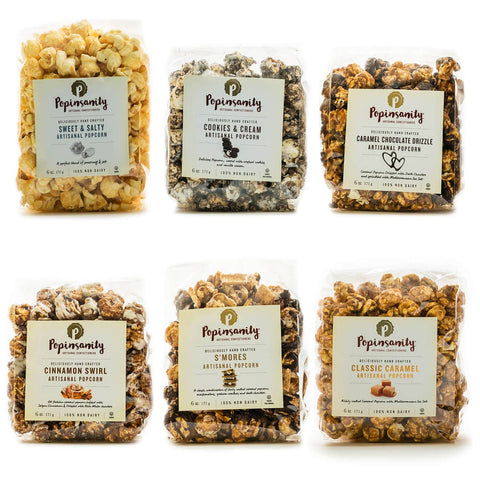The image is a photograph depicting six different varieties of gourmet popcorn, packaged in clear bags for retail sale. The brand name, somewhat difficult to decipher, appears to be "Popinsanity." Each bag showcases a distinct flavor with small, unique logos corresponding to each type. 

- Top left: Sweet and Salty, possibly denoted by a salt and sugar icon.
- Top middle: Cookies and Cream, distinguished by an Oreo-like illustration.
- Top right: Caramel Chocolate Drizzle, identifiable by its double heart symbol.
- Bottom left: Cinnamon Swirl, marked by a cinnamon roll graphic.
- Bottom middle: S'mores, represented by a s’mores symbol.
- Bottom right: Classic Caramel.

The popcorn flavors display a variety of colors, primarily browns and yellows, making them appear delicious and visually appealing.